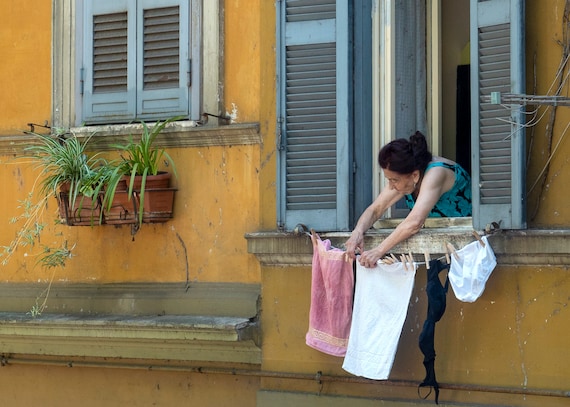The image captures an elderly woman in a blue tank top with her dark hair tied in a bun, stretching out of a window to hang laundry in a European, possibly Spanish setting. The old building features a yellowed wall and distinctive baby blue wooden blinds, with the upper shutters closed and the lower ones open. The woman uses a clothesline strung between the blinds to hang various items including a pink towel, a white towel, a white undergarment, and a black piece of clothing, all secured with clothespins. A terracotta hanging pot with lush green plants adorns the far left of the image, affixed to the wall below another smaller window with closed shutters. On the far right, visible cables run into the home, adding to the quaint, slightly rundown ambiance of the scene.